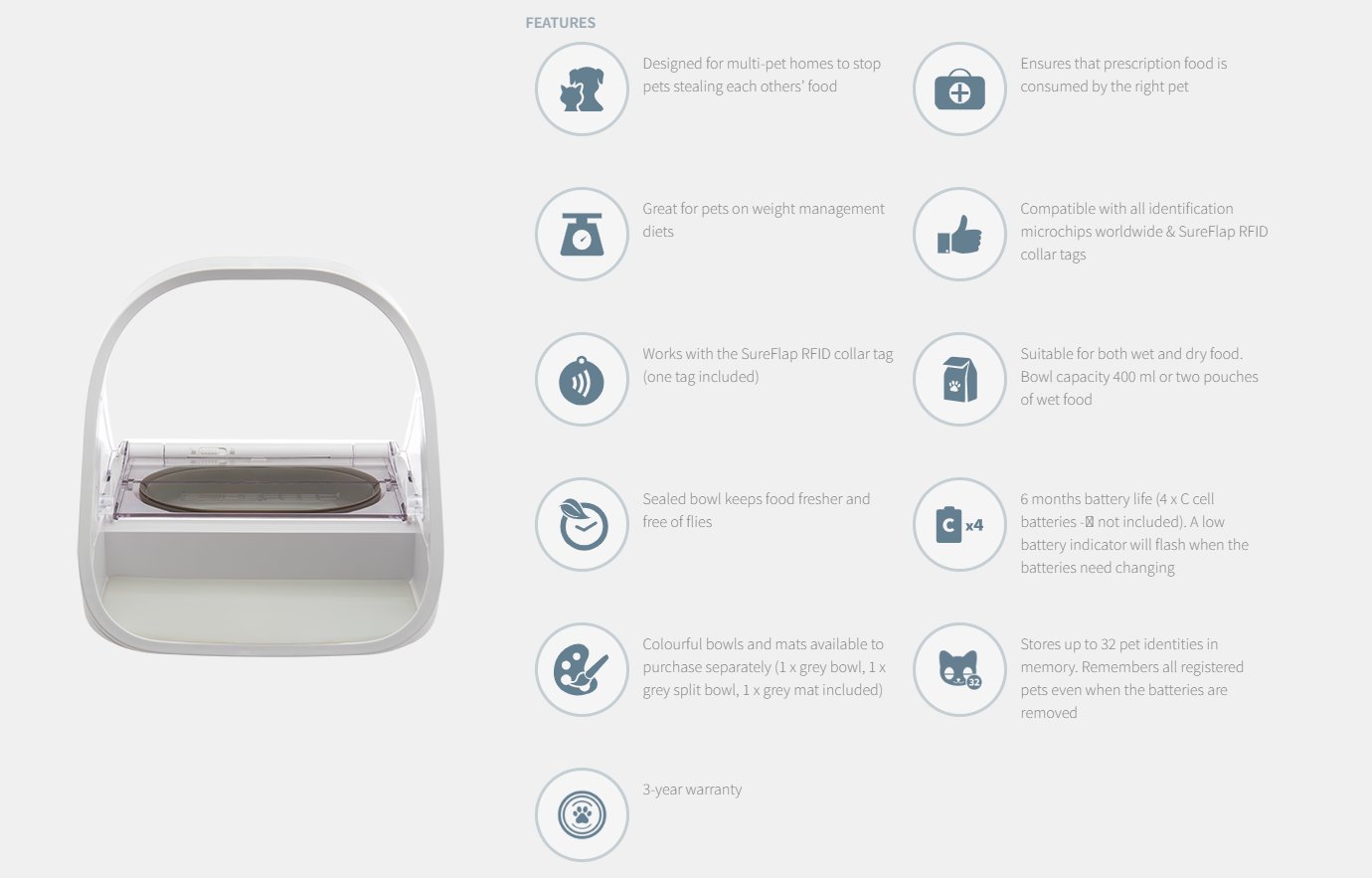Presented on a sleek grey background, this features page showcases a smart automatic dog feeder with a detailed breakdown of its capabilities. To the left, a high-resolution product image prominently displays the innovative feeder. On the right, the word "Features" is boldly positioned at the top center. Beneath it are several informative icons, each accompanied by a concise description:

1. **Multi-Pet Homes**: A circular icon depicts the silhouettes of a dog and a cat, indicating that the feeder is designed to prevent pets from stealing each other's food, ideal for multi-pet households.
   
2. **Weight Management**: A scale icon highlights the feeder’s suitability for pets on weight management diets, ensuring controlled portion sizes.

3. **RFID Collar Tags Compatibility**: An icon of an RFID tag signifies that the feeder works with secure tap RFID collar tags (tag not included), seamlessly integrating with your pets' accessories.

4. **Freshness Guaranteed**: An icon of a clock emphasizes that the bowl keeps food fresher and free from flies, promising a cleaner and healthier feeding experience.

Additional icons represent further key claims, each providing valuable insights into the feeder’s comprehensive feature set.